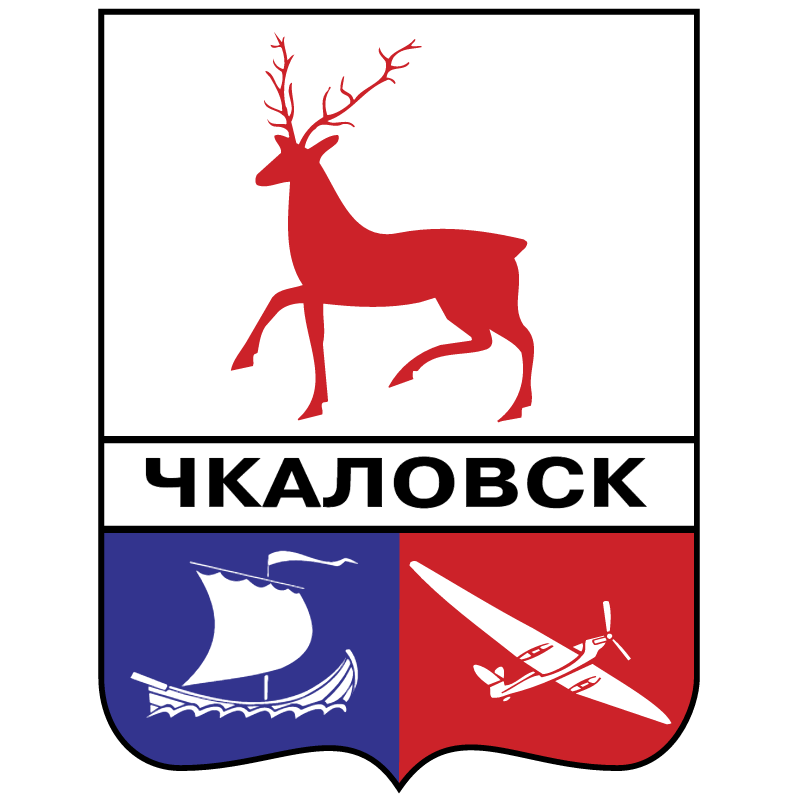The image depicts a distinctive coat of arms, likely representing a district in Russia, featuring a blend of symbolic elements and Cyrillic text. The banner-like emblem showcases a striking black border that shapes into a square at the top and rounds down to a pointed confluence at the bottom. Dominating the top portion is a red antlered deer, centered against a white background, symbolizing perhaps the region's native fauna or heritage. Directly beneath this, in bold black Cyrillic letters, is the word "Чкаловск," translatable to "Chkalovsk." This central text is prominently displayed. The lower section of the emblem is divided into two distinct parts: the left side with a white Viking-style sailboat set against a blue background, and the right side with a white single-engine plane on a red background, each illustrating the region’s maritime and aviation links. The harmonious arrangement and vivid color palette of black, white, red, and blue establish this emblem as a notable symbol of the Chkalovsk district, merging cultural and historical elements in a visually cohesive manner.